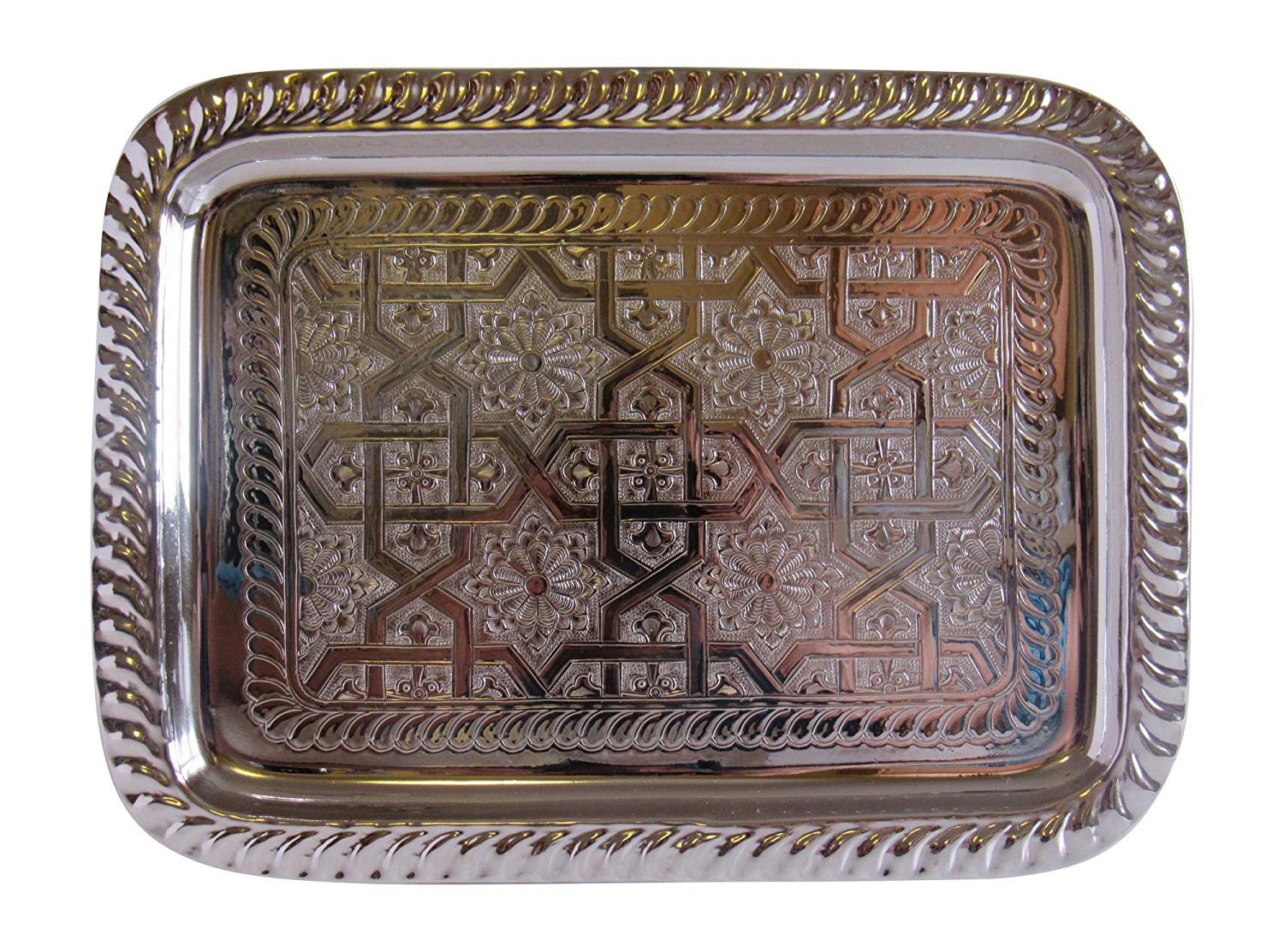This photograph captures an ornate silver and gold rectangular platter, taken from an overhead perspective. The platter features rounded corners and an outer ribbed edge that is slightly raised from the center. Inside this outer edge lies a smooth rectangular area, enclosed by another ribbed border. This middle section is lavishly decorated with a series of intricate etched designs, including four prominent star-like patterns resembling mandalas, interspersed with smaller ornamental details. The overall craftsmanship showcases a blend of metallic hues, giving the platter an elegant and intricate appearance.